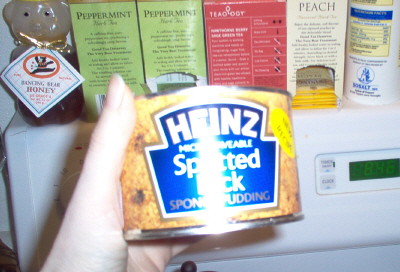A person holds up a can in their left hand, prominently displaying the label. The can is branded "Heinz," spelled out in white letters. The bottom part of the label has words that are obscured by a bright white light. In the background, a white washing machine is visible, positioned slightly behind the person's hand. The washing machine features a knob on the left side and a digital display glowing green on the right, accompanied by some labels to the left of the screen.